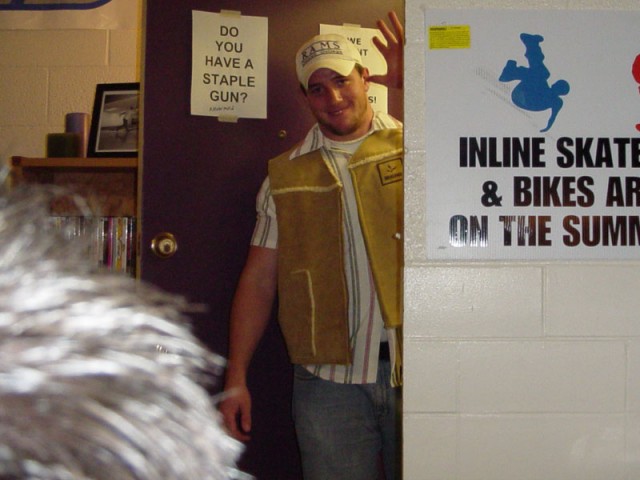This is a detailed photographic image taken indoors. It captures a white man standing and slightly waving at the camera, positioned in the doorway of what appears to be an office. The door behind him, made of brown wood, has a white sign taped to it that reads, "Do you have a staple gun?" The man, who has a short beard and is smiling warmly, is wearing a white baseball cap with the word "Rams" on it, a brown vest over a striped shirt featuring purple and gray stripes on a white background, and likely blue jeans. To the right of the image, mounted on a white concrete wall, is a sign with black print and a blue skater outline, reading "Inline Skate and Bikes are on the SUM." The bottom left corner is slightly obscured by what appears to be the hair of another person. In the background, which also has the same white concrete walls, there is a bookshelf adorned with a framed photo.